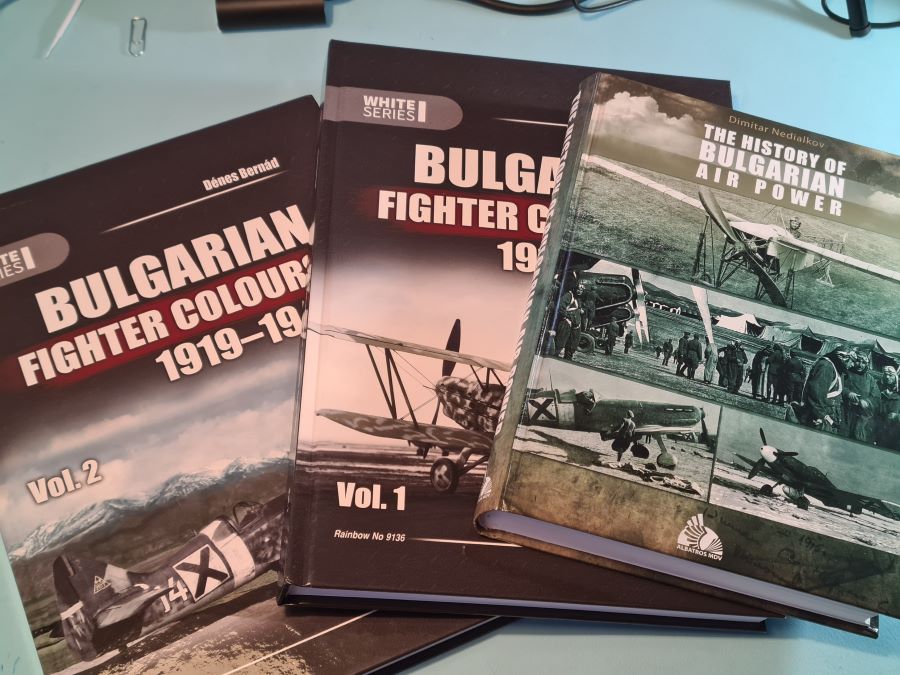The image depicts three hardcover books fanned out on a white desk or table, each focusing on Bulgarian air power and fighter colors from the early 1900s. The leftmost book, partially obscured, is titled "Bulgarian Fighter Colors 1919-19--" with the remaining date not visible and is labeled as Volume 2. The center book, identified as Volume 1, also titled "Bulgarian Fighter Colors," also has its dates partially obscured. The rightmost, fully visible book is "The History of Bulgarian Air Power" by Dimitry Nadevlov, featuring multiple black and white photographs of airplanes and aircraft carriers on its cover. At the top of the image, various office supplies including a silver paper clip, a black charging cable, and the edge of eyeglasses are partially visible.